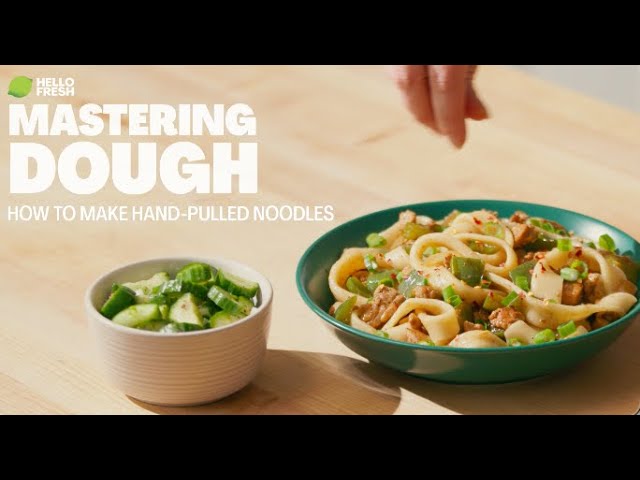This image is a promotional screenshot for Hello Fresh, showcasing their video titled "Mastering Dough: How to Make Hand-Pulled Noodles," as indicated by the white text in the top left corner beside a green lime logo. The scene is set on a light wooden countertop featuring two distinct bowls of food. On the left, there's a small white ceramic bowl with ridges, containing sliced cucumbers or possibly bitter melon. On the right, a shallow, round, turquoise bowl holds a complete noodle meal, garnished with fresh herbs, chopped onion greens, and slices of meat. A hand extends from the top right, appearing to sprinkle a garnish over the noodle dish, adding an interactive element to the preparation scene.